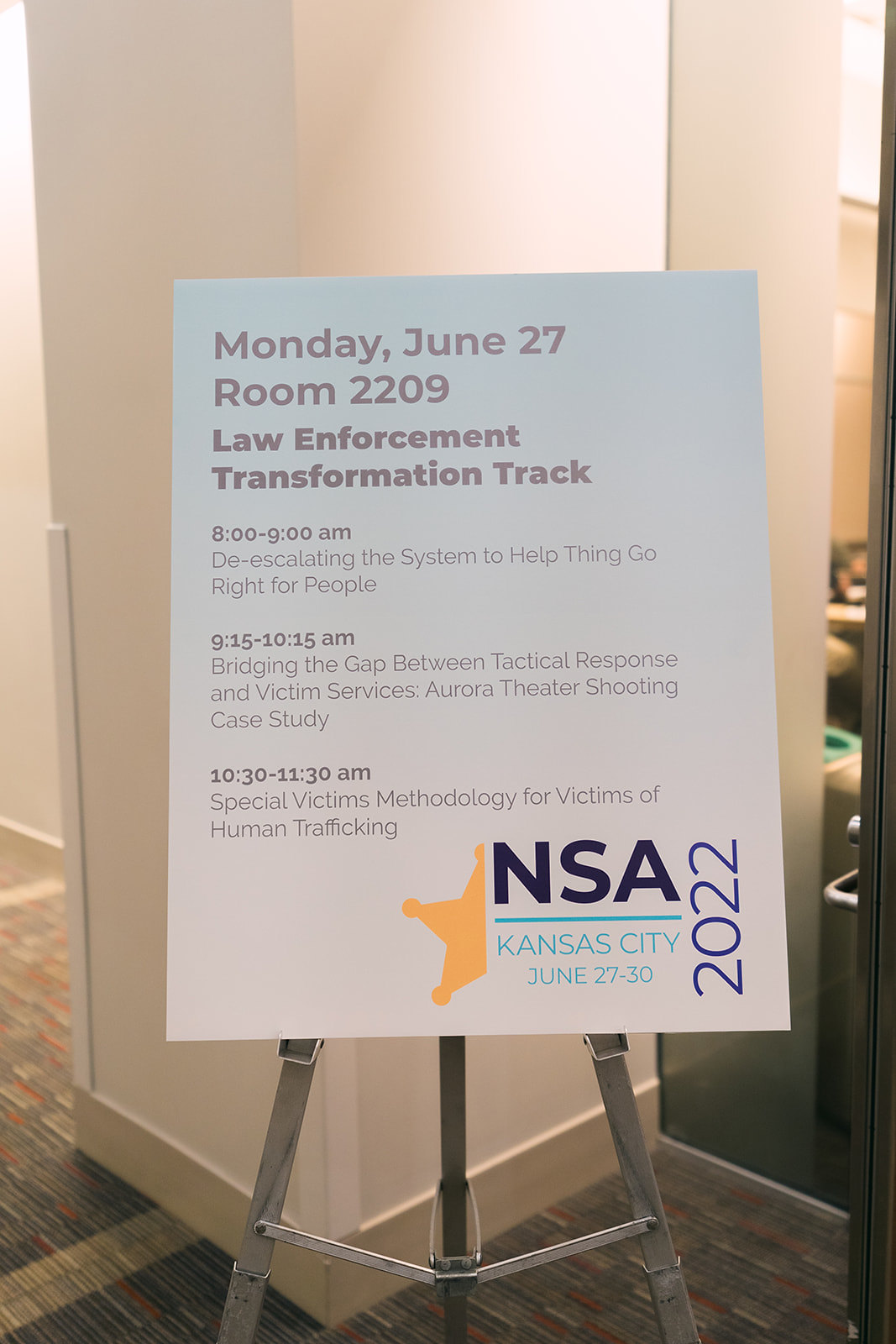The image features a detailed poster displayed on an easel stand in what appears to be a conference room setting. The poster is centered, showcasing the following information in black text on a white background: 

- **Monday, June 27th, Room 2209**
  - **8:00-9:00am:** "De-escalating the System to Help Things Go Right for People"
  - **9:15-10:15am:** "Bridging the Gap Between Tactical Response and Victim Services or Aurora Teacher Theater Shooting Case Study"
  - **10:30-11:30am:** "Special Victims Methodology for Victims of Human Trafficking"
- **NSA, Kansas City, June 27-30, 2022** 

The header features the emblem of a sheriff's star partially visible next to the NSA text. The poster is accented with colors - gold, dark blue, light blue, regular blue, and black text, set against a light blue-white backdrop. The easel is gray metal and stands on a carpet patterned in shades of blue, red, and tan. The backdrop is a cream-white wall, indicative of a hotel or conference room setup, highlighting the Law Enforcement Transformation Track at a convention in Kansas City.